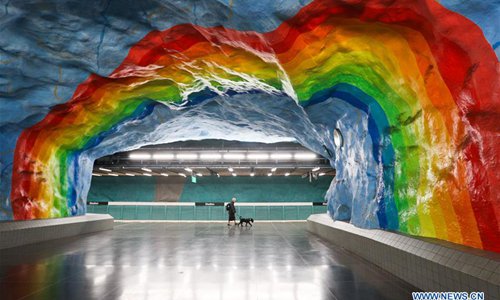In this intriguing and abstract image, a person, seemingly a woman given the hint of a skirt, walks a black, medium-sized dog on a leash. They traverse the middle distance of what appears to be a tunnel or an open, expansive hallway. The floor is dark gray, polished, and highly reflective, capturing the play of light across its surface. The tunnel or hallway is adorned with a colorful, uneven rainbow design that arches from the left side, above the figures, and down to the right. This rainbow features a spectrum of colors: red, orange, yellow, green, darker green, blue, and darker blue.

On either side of the hallway, rails are visible, and ahead, there's a row of lights suggesting the entrance to another space, possibly a stadium or a museum. The end of the hallway features a horizontal bar in front of a blue tiled wall with a light row above it. The sky above the rainbow varies in blue shades, creating a dynamic visual effect with its crinkly texture. The bottom right corner of the image is marked with "www.news.cn." This captivating scene blends an architectural structure with artistic and whimsical elements, creating a visually stimulating environment.